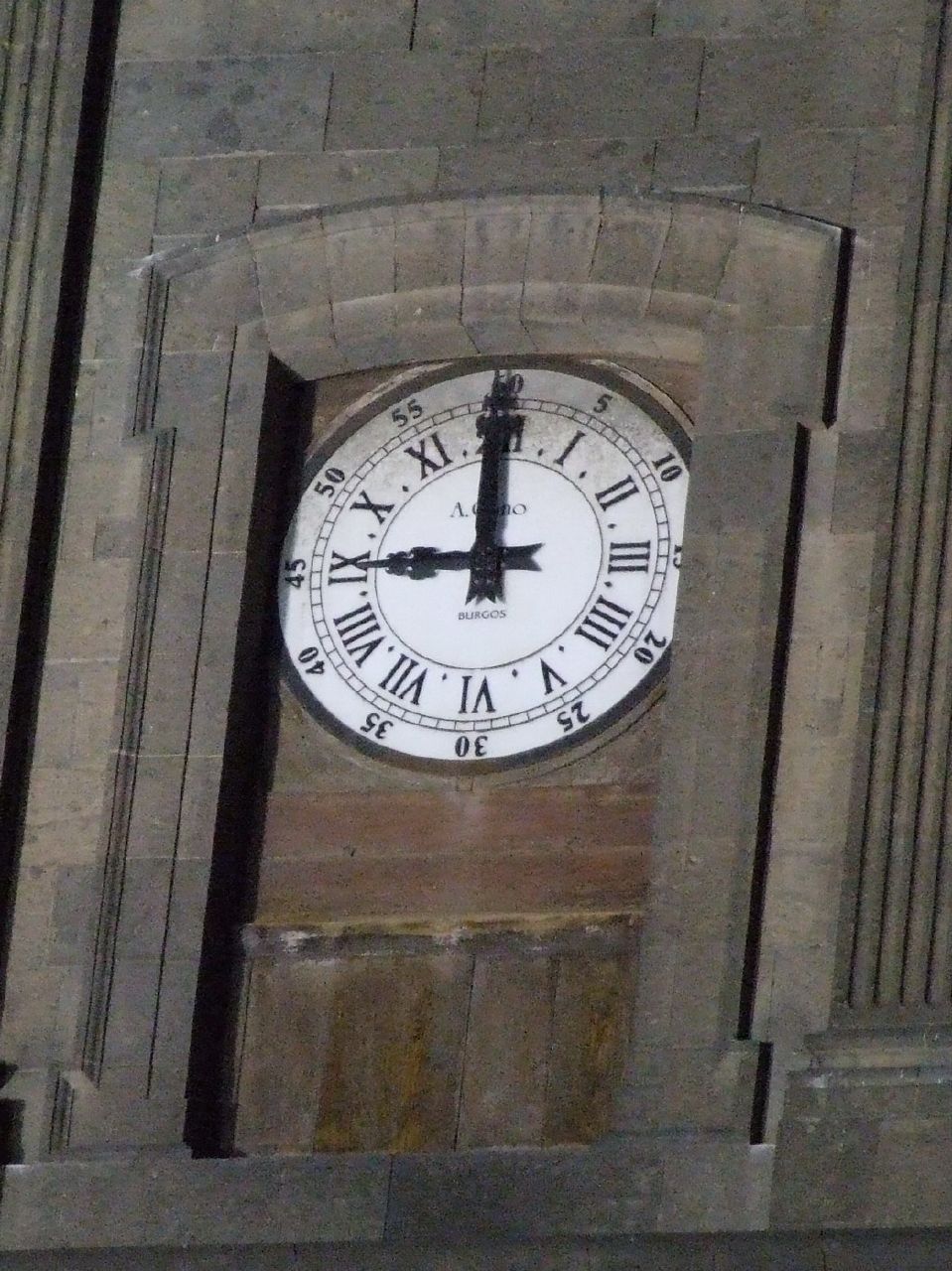The image depicts a section of an old stone structure, possibly part of a building or a bell tower, characterized by its gray, rectangular-shaped stones. The wall features a distinct rectangular inset in the middle, where the stones are vertically oriented, contrasting with the horizontally positioned stones in the surrounding sections. Within this inset, there is a smaller section made of red bricks, adding a layer of visual interest. A large, circular clock with a predominantly white face and black Roman numerals is mounted in the center of this red brick section. The clock also includes regular numbers in increments of five around the outer edge. The black metal hands of the clock are positioned at nine and twelve, indicating the time as nine o'clock. The overall architecture and design elements suggest the structure is quite old.